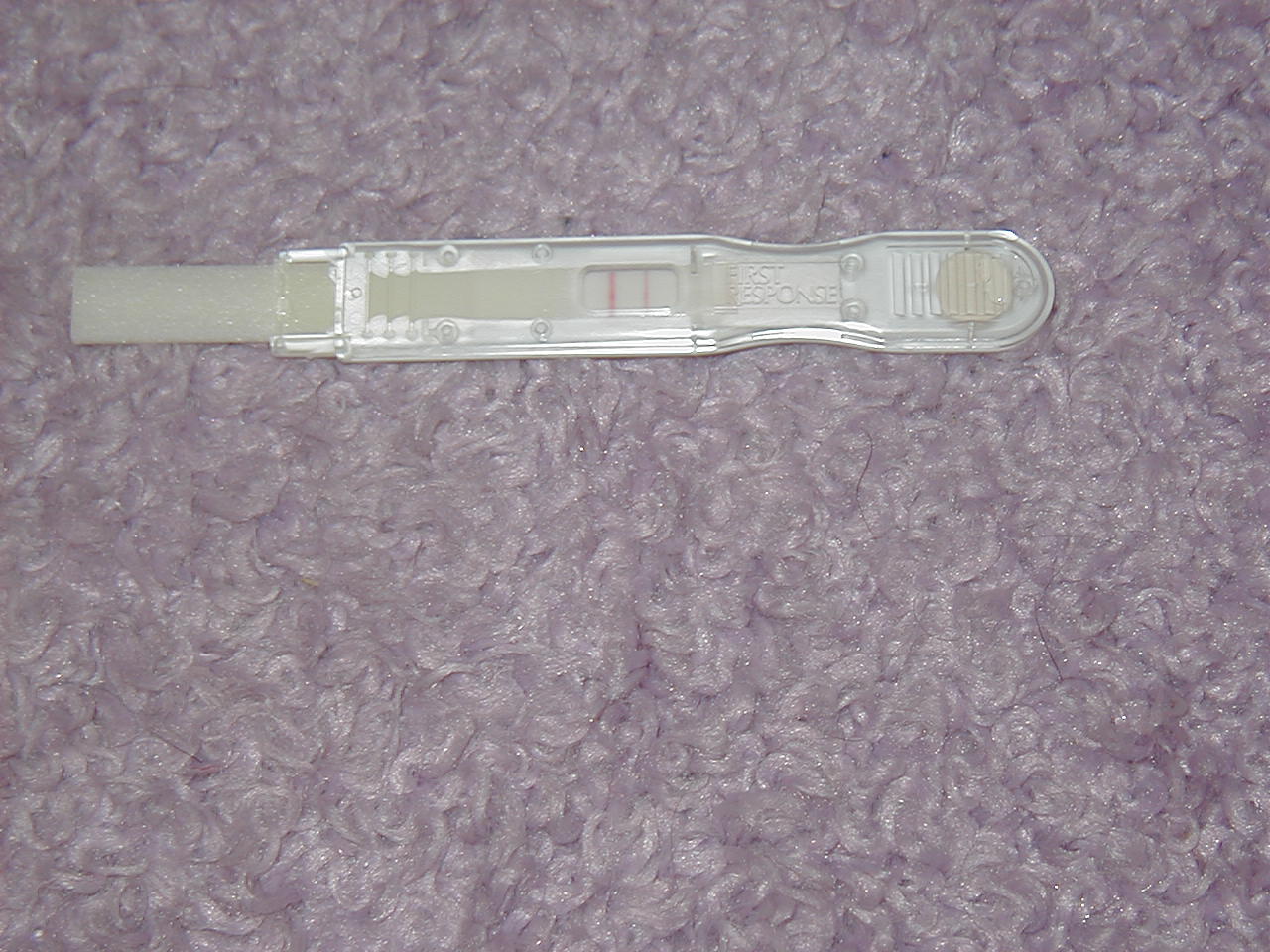In this well-lit photograph, a First Response pregnancy test is prominently displayed on a white-gray carpet. The carpet's texture features noticeable swirls and tufts, interspersed with small dark hairs and shiny, glitter-like areas that catch the light. Positioned towards the top center of the image, the test itself is a long, curved plastic device. One end of the test extends into a white foam or plastic component. The body of the test bears the text "First Response," and features ergonomic edges designed for easy handling. Clearly visible are two lines on the test indicator, signifying a positive result. The plastic casing of the test is held together by small, secure plastic connectors.